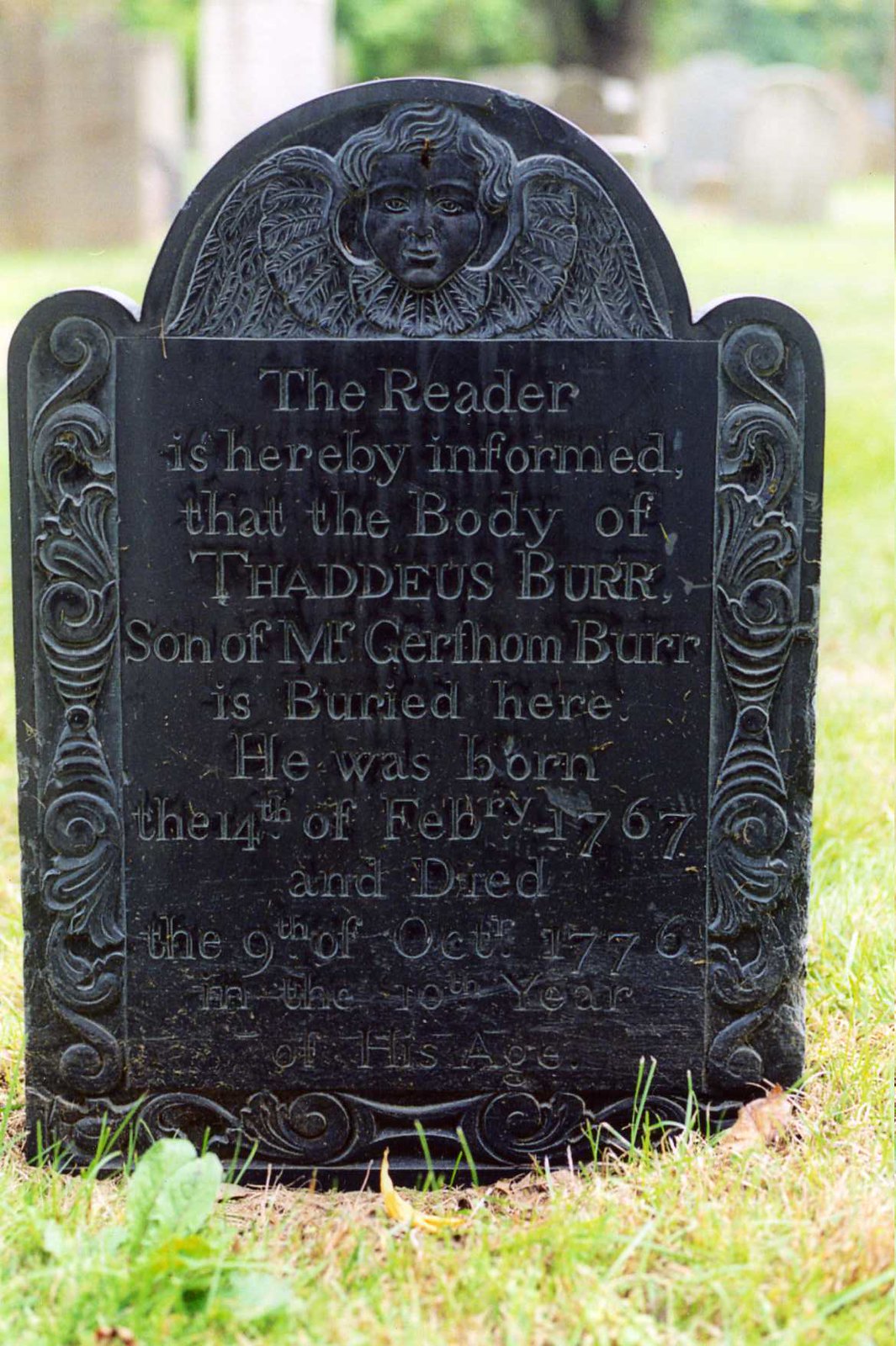The image is a zoom-in of a black stone grave, possibly made of granite or slate, featuring a half-dome shape at the top. At the upper part of the tombstone, there is a carved depiction of a childlike angel with two wings. The grave's surface is adorned with elaborate, ornate designs resembling paisley patterns on the right, left, and bottom edges. The inscription on the grave states, "the reader is hereby informed that the body of Thaddeus Burr, son of Mr. Gerhom Burr, is buried here. He was born on the 14th of February, 1767, and died on the 9th of October, 1776, in the 10th year of his age." The grave is set amidst green grass that appears quite bright, suggesting that it is a sunny day. Additionally, glasses surround the grave, adding to the intricate detail of the scene.